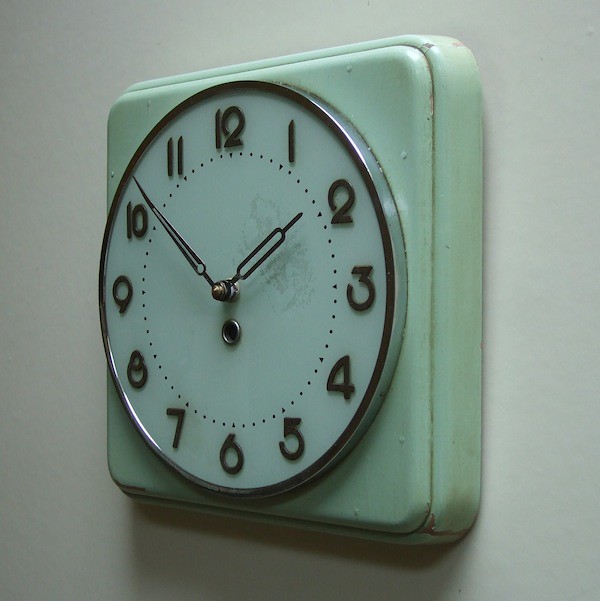The photograph captures a unique clock mounted on a white wall, seen from a diagonal angle that emphasizes its distinct design. The clock, an Amarillon model, features a perfectly round face encased within a mint green, square frame that has rounded edges. The green base displays signs of wear, with paint chipped away in spots, revealing a metallic construction beneath. Hints of rust and chipped paint attest to its age.

Encircling the clock face is a chrome border that slightly overlaps onto the dial's circumference, adding a sleek contrast to the weathered green body. The clock's face contains black numerals, arranged in a circular pattern from 1 to 12, and small dots marking the minutes. The hands of the clock, metallic and arched, show the time as 10:02, with the minute hand pointing just past the 10 and the hour hand nearing the 2. A small recess in the center of the face, below the hands, adds to the clock's detailed construction. In the background, the light gray wall casts a subtle shadow beneath the clock, further highlighting its vintage charm.